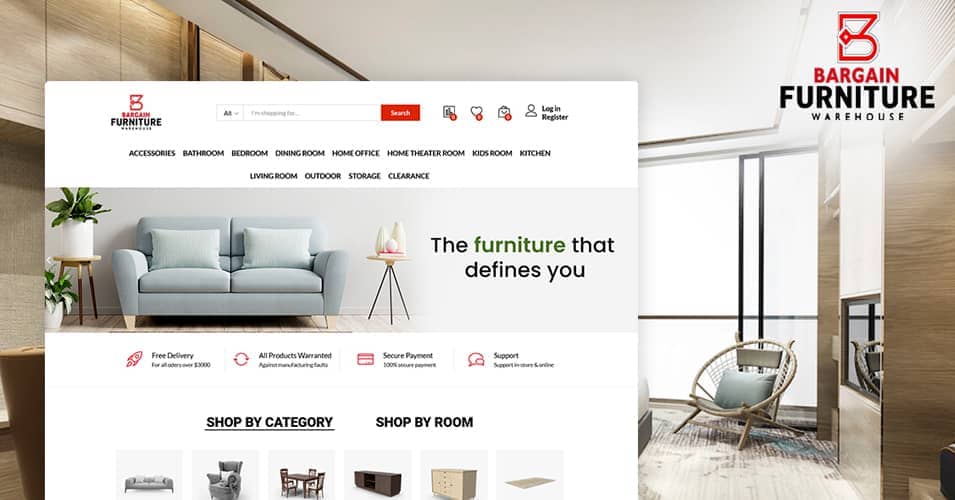**Detailed Descriptive Caption:**

The image is a left-to-right horizontal advertisement for a furniture store, designed for digital platforms such as webpages or emails and suitable for viewing on computers or smartphones. The background showcases a modernized living room with large windows letting in bright natural light. Prominently visible in the room is a wicker chair adorned with a blue pillow and a set of sleek cabinets in the background.

In the upper right corner, a logo featuring a small "B" symbol is present, followed by the text "Bargain" in red, "Furniture" in black, and "Warehouse" in smaller black font beneath it.

Overlaying this background is a sleek, white interface representing the store's webpage. At the top, there are several interactive elements: a search box, a heart icon, a shopping bag, and options to log in or register. Below these, several clickable icons categorize the store's offerings into sections such as Accessories, Bathroom, Bedroom, Dining Room, Home Office, Home Theater Room, Kids Room, Kitchen, Living Room, Outdoor, Storage, and Clearance.

The main focal point of the advertisement is a central image of a couch with the tagline "The Furniture That Defines You" beneath it. Additional promotional points highlighted include free delivery, all products guaranteed, secure payment, and support. Towards the bottom, users are invited to shop by category or room, with corresponding icons providing visual cues for ease of navigation.